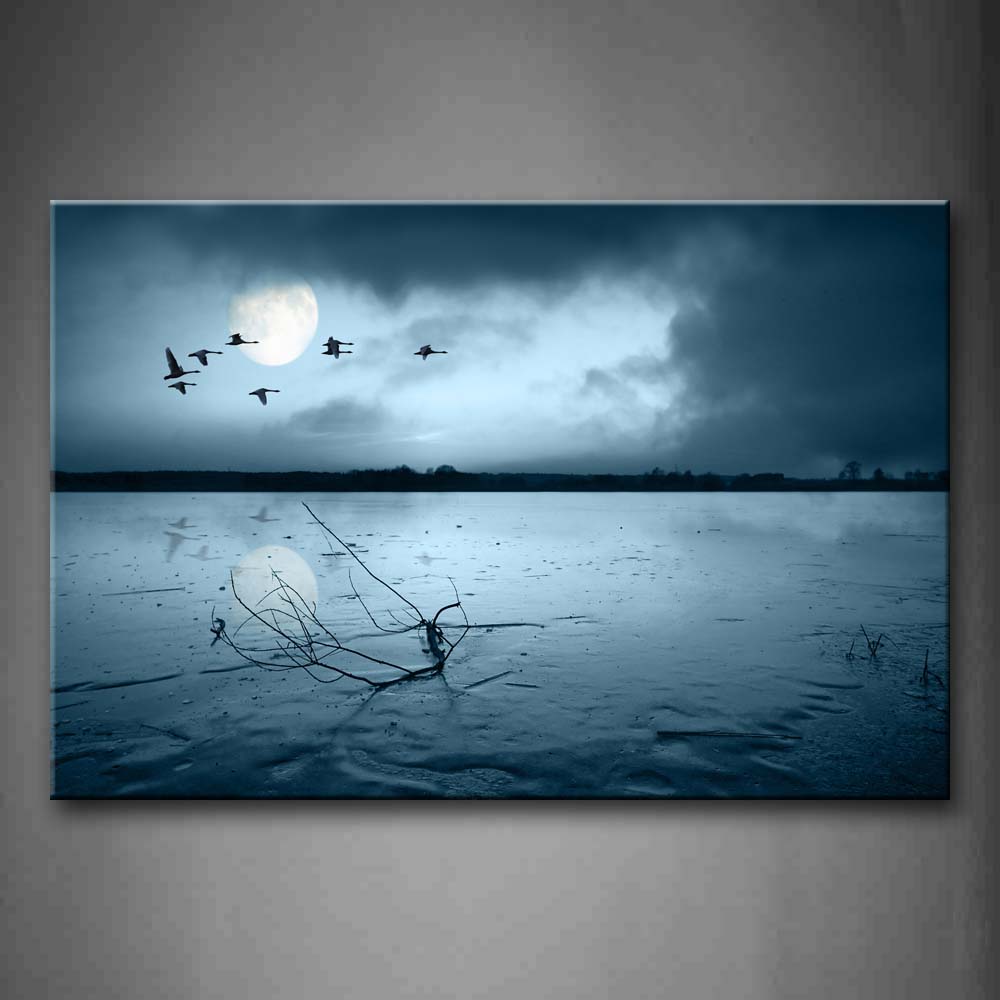This is a photograph of a painting, displayed on a gray wall with a light source illuminating its center. The painting is a horizontal rectangle, depicting an ominous and tranquil nocturnal scene over a still lake with dark blue water. Ripples on the water's surface suggest a recent evening rain, and reflections of birds flying overhead are visible. Towards the bottom left, a floating branch, colored dark blue due to the sky and water, juts out with multiple smaller branches. On the right, two plants emerge from the water's edge.

The background features a dark blue and black silhouette of trees and grass on the distant shoreline. A flock of eight birds, likely geese, flaps in formation from right to left across the sky, their black silhouettes contrasting against the night sky. To the right-hand side, the sky is filled with a mixture of dark gray and blue storm clouds. A moon with a white surface and gray blotches partially obscured by these clouds casts a faint, gloomy light, which is also reflected on the water below, enhancing the painting's somber and grim atmosphere.